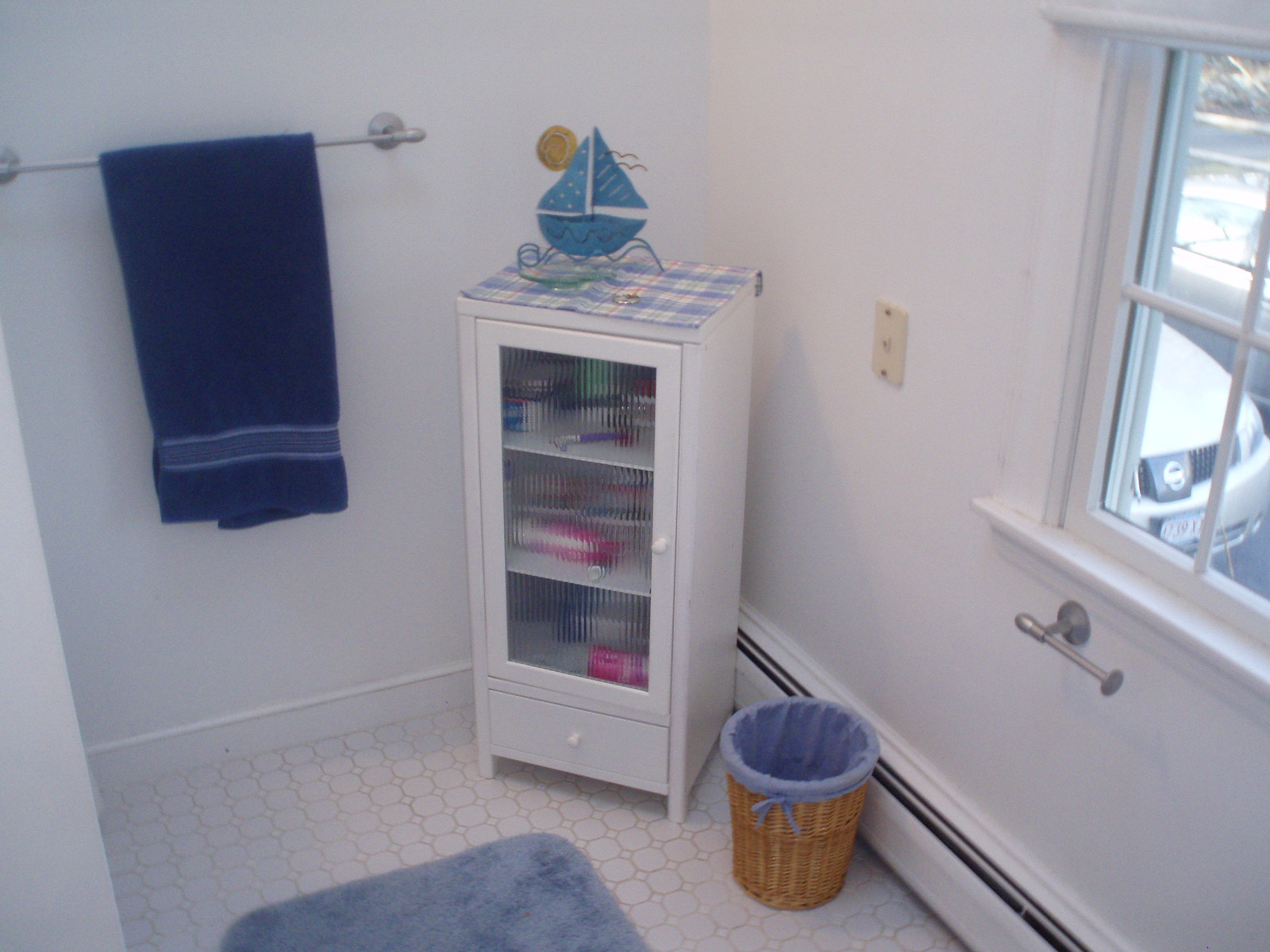A meticulously organized bathroom featuring small tile flooring. The scene captures a cozy blue mat placed just outside a spacious shower. Adjacent to it, a matching blue towel drapes neatly from a sleek rack. A prominent little cabinet with semi-transparent glass doors, adorned with subtle vertical grooves, stands beside it; though the items inside remain a bit obscured by the glass, adding an air of mystery. Atop this cabinet sits a quaint mat as well as an artistic sailboat, possibly a charming craft by a child. 

A wicker wastebasket with a neatly lined blue trash bag adds to the room's cohesive color theme, emphasizing the abundant blue accents. The pristine white walls enhance the room's brightness, and a window on the right side bathes the space in natural light. Through the window, a parked silver sedan is visible, grounding the bathroom in its real-world setting. Despite the room's lived-in feel, everything is immaculately clean, save for an empty toilet paper holder waiting to be refilled.